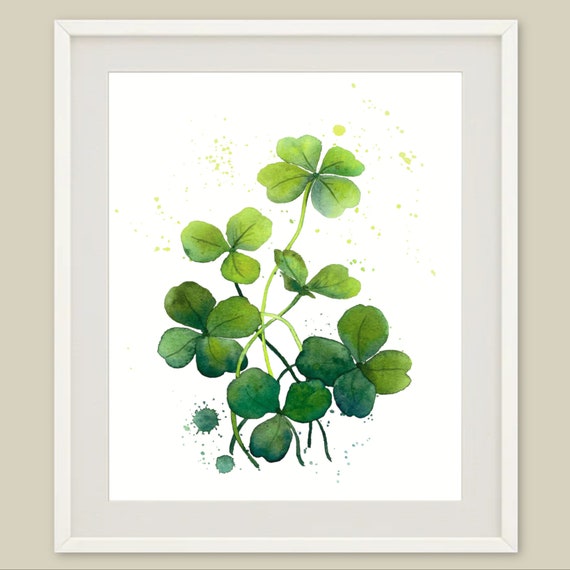The rectangular image, slightly taller than it is wide, depicts a framed picture set against a beige background. The frame itself is a soft off-white color with a gray inner border, enclosing a white canvas. On this white background, there's a delicate arrangement of six green clovers, some with three leaves and others with four. These clovers show a gradient of greens, with lighter shades at the top progressing to darker greens at the bottom, and slender stems are visible extending from each plant. Interspersed among the clovers are splatters of green in varying shades, mirroring the gradient effect from light to dark. Despite a mention of lavender hues in one description, the predominant colors in the image are white, gray, and green. The overall visual effect is clear and detailed, presenting a charming and simple botanical display.